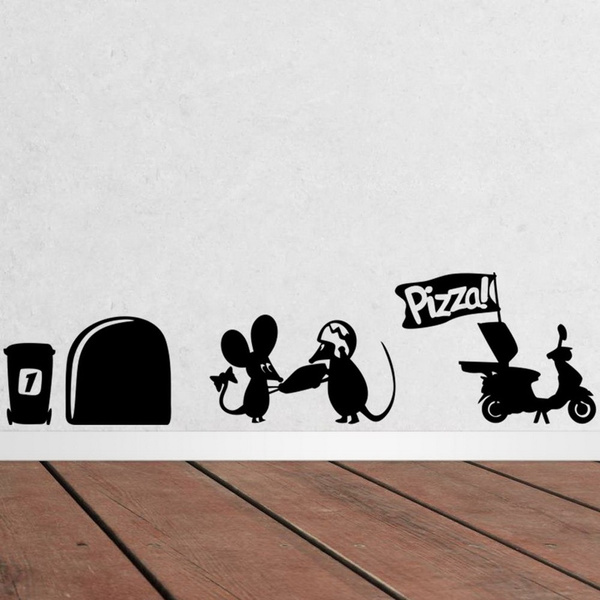The image showcases an artistic drawing on a grayish-blue wall with a clean, white border at the bottom. Below the border, there's a floor made up of thin, reddish-brown wooden panels arranged in rows. The wall features a playful scene rendered in black and white. On the far left, there's a small black garbage can labeled with the number "1." Next to it is an oval-shaped mouse hole reminiscent of old cartoons. Standing nearby are two mice: the one on the left has a bow on its tail, and the one on the right, wearing a motorcycle helmet, is handing over a pizza box. To the right of these mice, there's a motorcycle complete with a flag that says "PIZZA." The entire setting exudes a charming and whimsical atmosphere, captured with bright and clear visual detail.